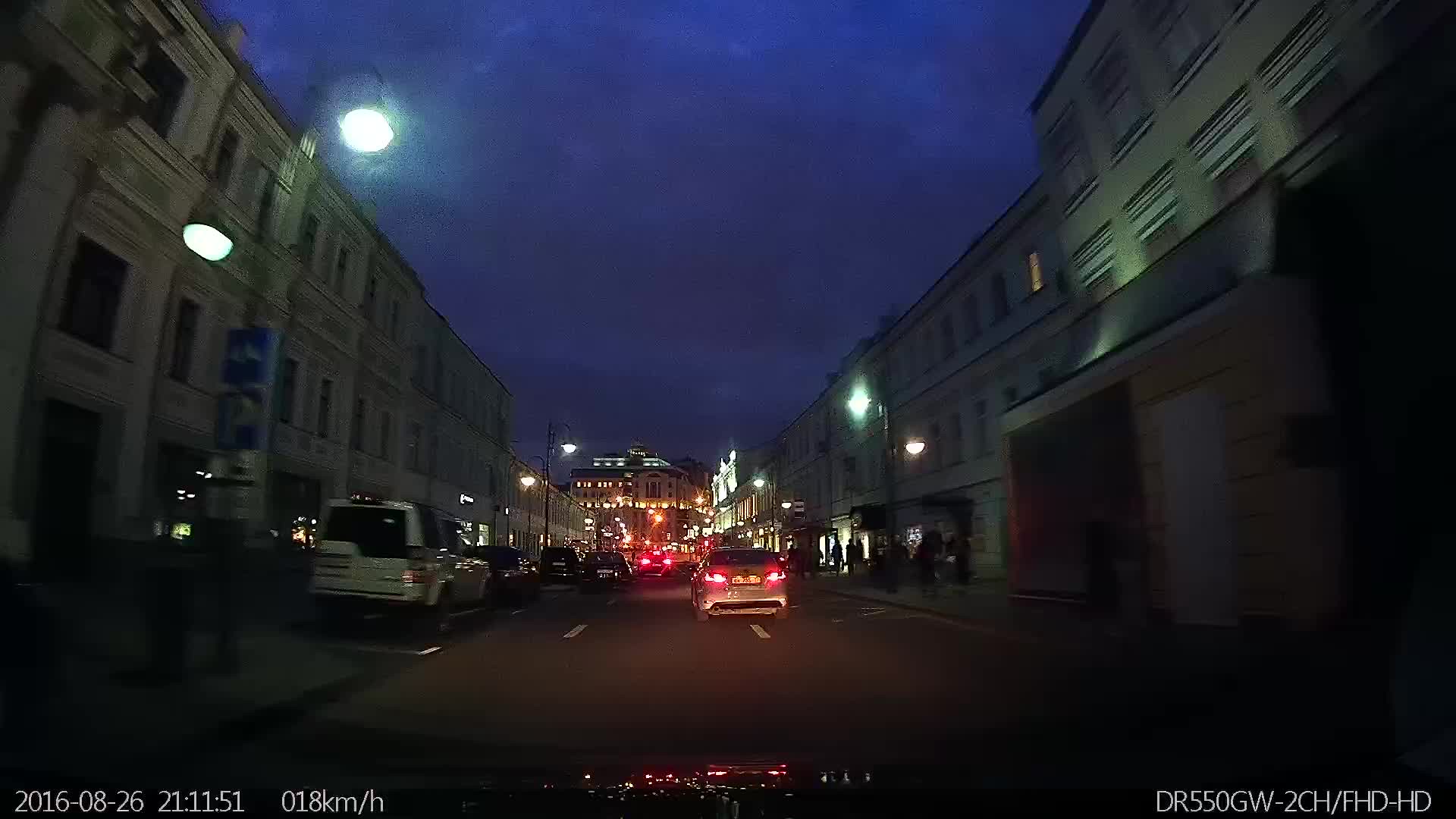This photo, captured from a dashboard camera at night, is blurry and pixelated but provides a detailed view of an urban street. The scene depicts a two- to three-lane road with parked cars lining the left side. In the center lane, a car with its brake lights on is visible, seemingly straddling two lanes. The street is flanked by three-story buildings that have a retro, possibly European, architectural style, with street lamps illuminating the scene due to the cloudy, overcast sky. In the distance, a large building can be seen. Beneath the scene, a time and date stamp reads "2016-08-26, 21:11:51," and indicates the vehicle's speed as "0.18 kilometers per hour." The make and model of the dash cam, "DR55OGW-2CH-FHD-HD," are displayed in the bottom right corner.